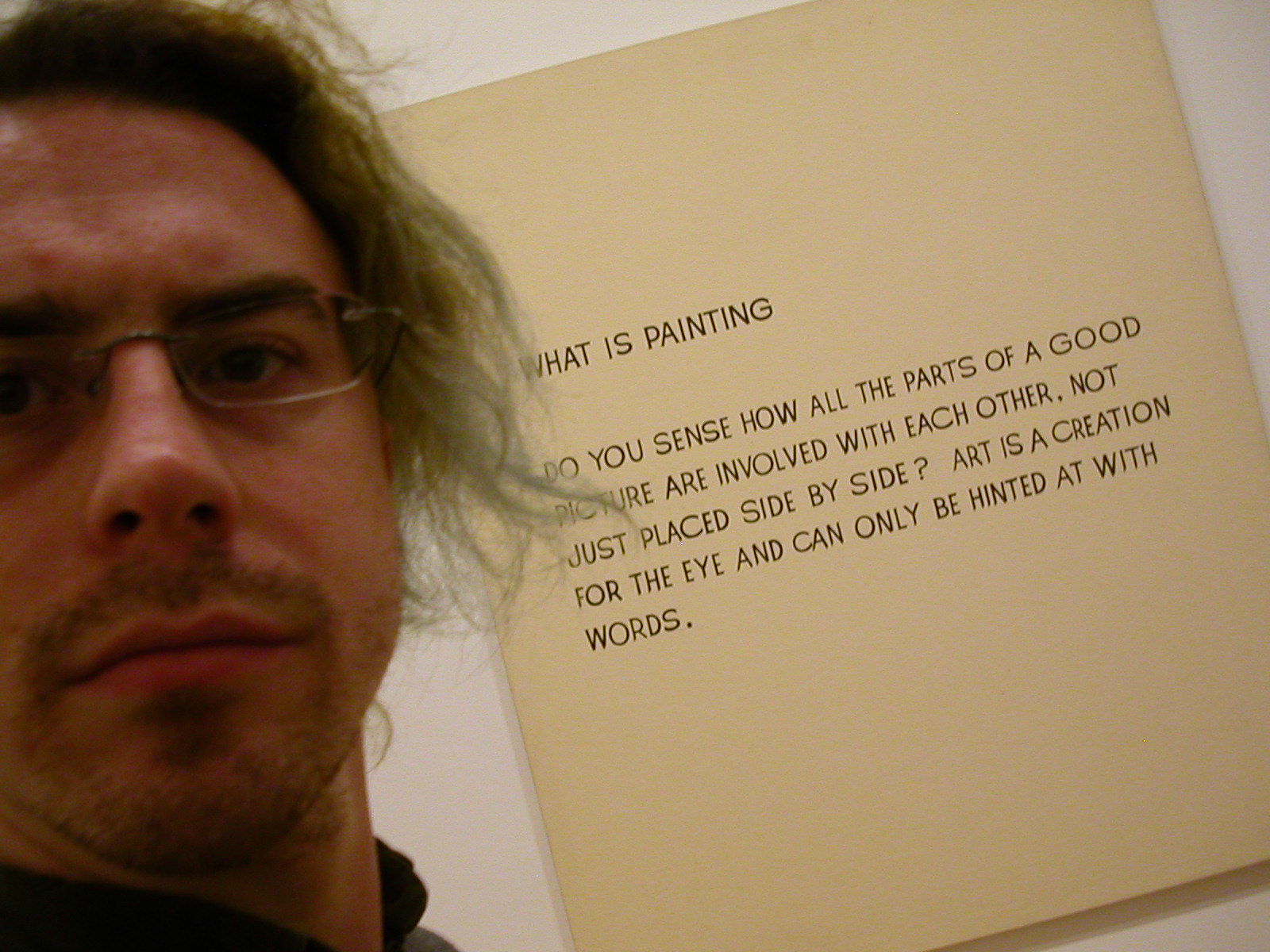The photograph features a close-up of a presumably unshaven artist on the left third of the image. The man, wearing rimless glasses, displays straggly, unkempt blonde hair while sporting a bit more than a five-o'clock shadow. His expressive brown eyes, one of which is slightly cut off by the cropping of the image, engage the viewer. Adjacent to him on the right side, tilted at an angle of about 40 degrees, there is a beige placard with a thought-provoking message in black text: "What is Painting? Do you sense how all the parts of a good picture are involved with each other? Not just placed side by side. Art is a creation for the eye and can only be hinted at with words." The background of the image is a subdued pale gray or white, suggesting an art gallery, museum exhibit, or artist’s show setting. The juxtaposition of the artist's intense gaze and the reflective placard invites viewers to ponder the interconnectedness of art’s elements.